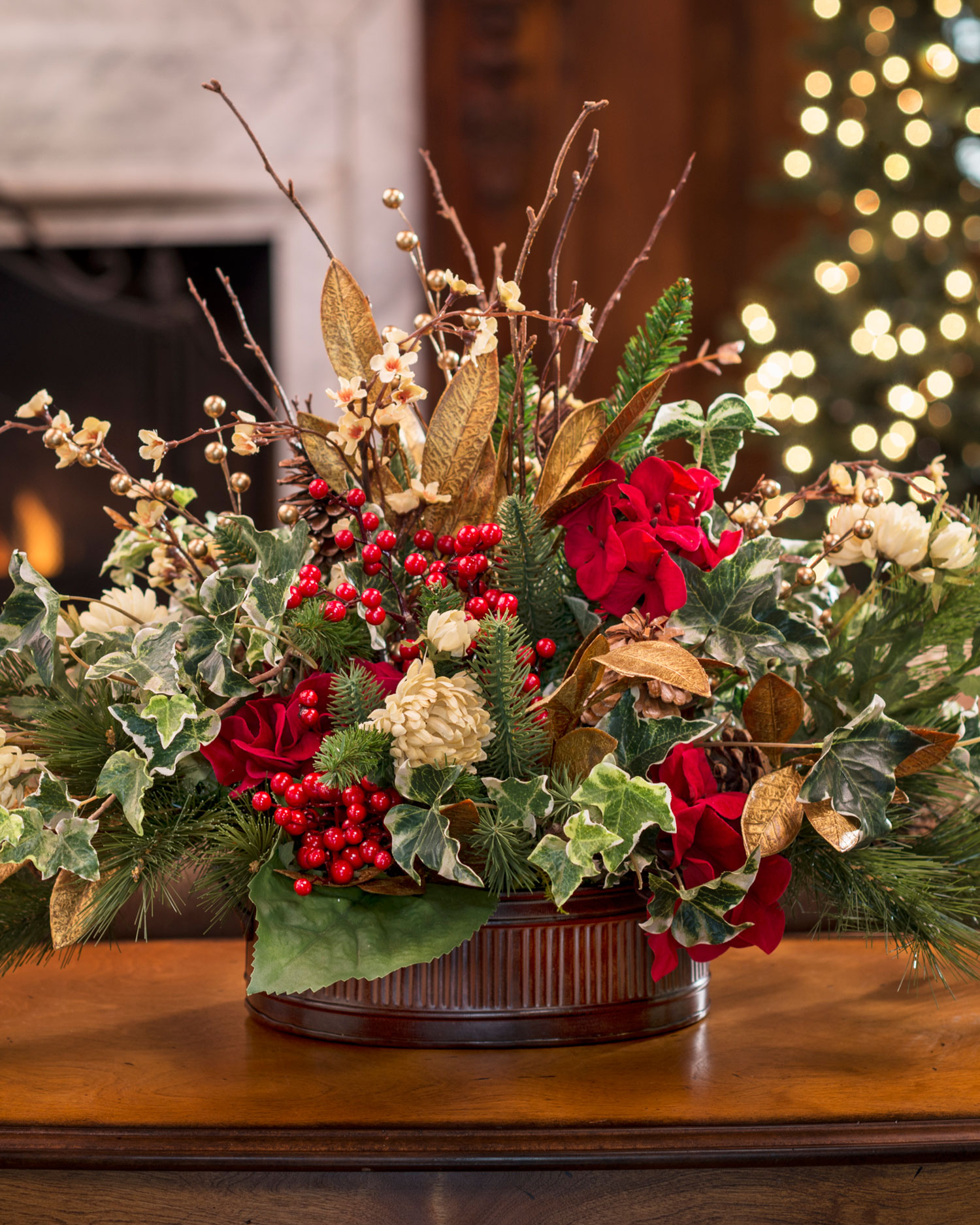This color photograph captures a charming Christmas bouquet set on a honey-brown wooden table. The arrangement is nestled in a round cherry wood container, adding a rustic touch. The bouquet is a festive mix of greenery, including green ivy and pine, interspersed with red and gold berries, white and beige flowers, brown and gold leaves, and twigs that add a natural element. Behind the arrangement, to the left, stands a white fireplace with a glowing fire. In the background, there is a brown wall, and in the upper right-hand corner, a decorated Christmas tree adorned with white and yellow lights peeks into view. The scene is beautifully framed by the white doorway on the left, where a warm yellow light glows in the distance, enhancing the cozy Christmas ambiance.